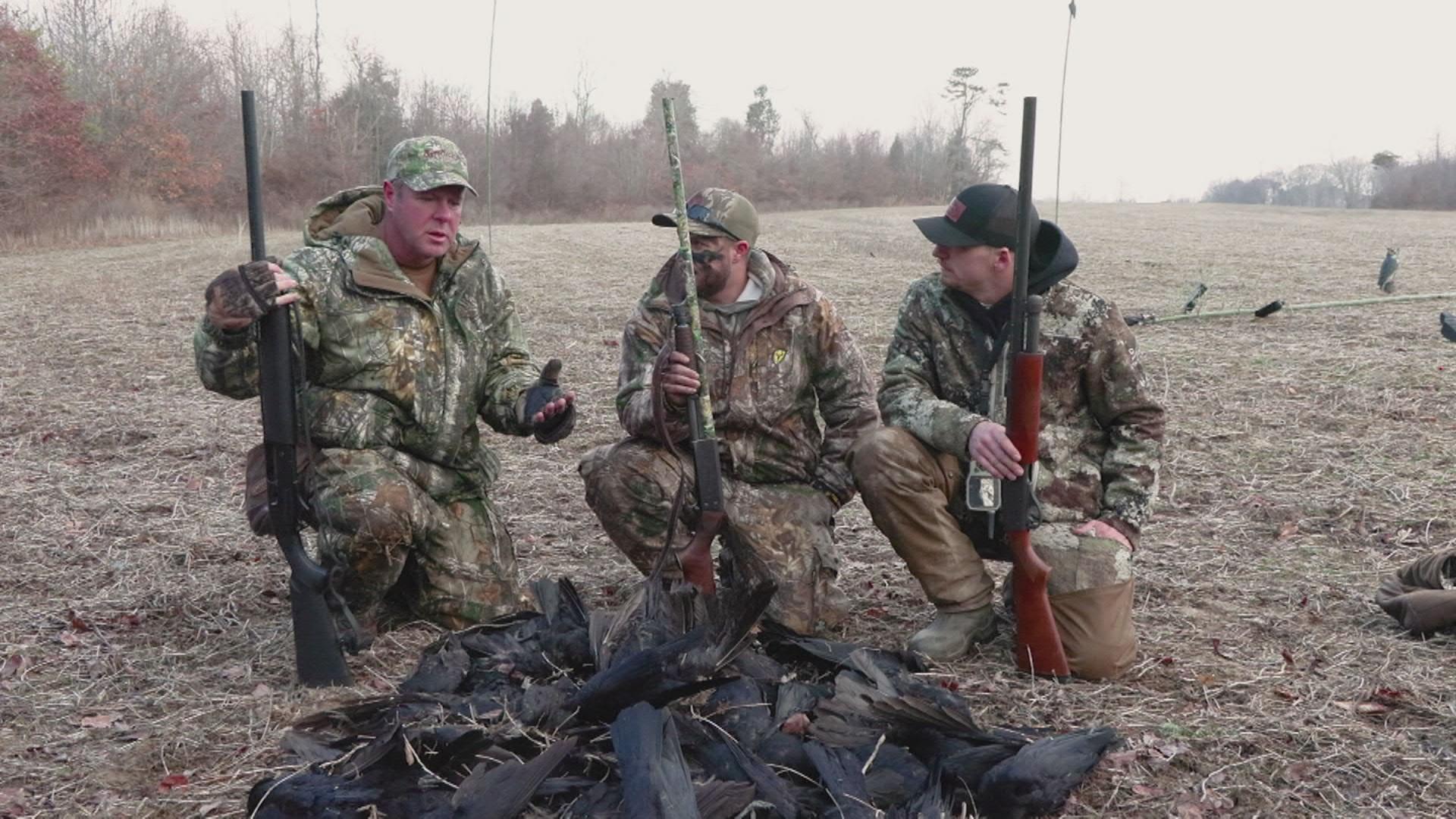In this image, three hunters are down on one knee in a vast, open field with brown, dead grass under a cloudy, white sky. They are clad in typical green and brown camouflage jackets and two of them wear matching camouflage hats, while the third sports a black hat with a red logo. Each man holds a long rifle, pointed skyward, showcasing their hunting gear. In front of them lies a dark pile, likely consisting of birds or ducks they have successfully hunted. Behind them is a line of trees, some adorned with red and green leaves. They appear to be posing proudly, possibly after extinguishing a campfire, as one man converses with the others. The serene backdrop underlines their readiness to continue their hunting excursion.